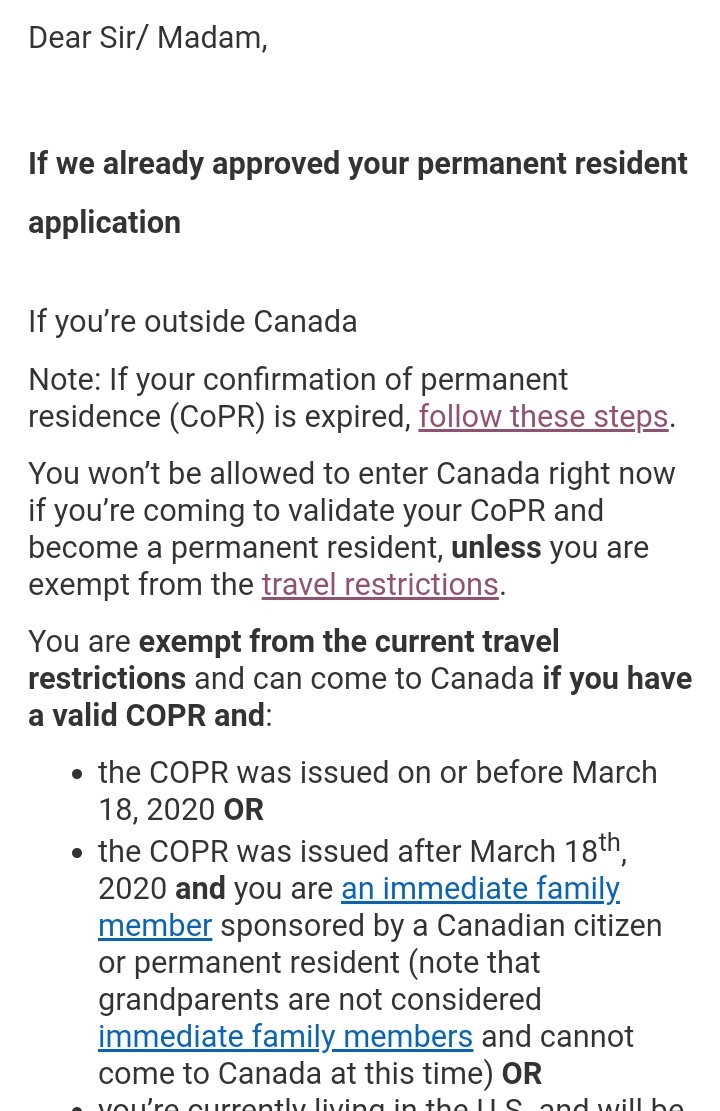The image displays a page containing detailed information about the approval process and travel restrictions for permanent resident applications to Canada. At the top, in bold text, it reads:

"Dear Sir/Madam, if we have already approved your permanent resident application..."

Following this, there's a note for individuals currently outside Canada:

"If your Confirmation of Permanent Residence (CoPR) is expired, follow these steps."

In purple, underlined text, it instructs to:

"You won't be allowed to enter Canada right now if you're coming to validate your CoPR and become a permanent resident unless you are exempt from the travel restrictions. You are exempt from the current travel restrictions and can come to Canada if you have a valid CoPR and..."

The conditions are listed with bullet points:
1. The CoPR was issued on or before March 18, 2020, or
2. The CoPR was issued after March 18, 2020, and you are an immediate family member (in purple underline) sponsored by a Canadian citizen or permanent resident. Note that grandparents are not considered immediate family members and cannot come to Canada at this time.

The information further intended to explain the third bullet point is cut off in the image.